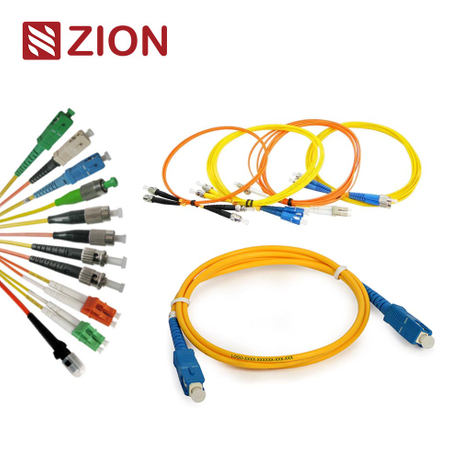The image features a white background with "Zion" displayed in the upper left corner in maroon colored font. On the left side, there is an assortment of various electrical cords and wires in an array of colors and designs. The cords include shades of green, gray, blue, red, black, orange, yellow, and pink. Some cords have metallic parts, resembling ethernet cable ends, while others feature multiple colors and patterns. Among these, there are also distinctive cord plugs in blue and green, with some in a darker turquoise shade. These cords appear to be part of a collection presented by the company Zion, which showcases a wide selection of their available electrical wires, each with its unique design and color combination.